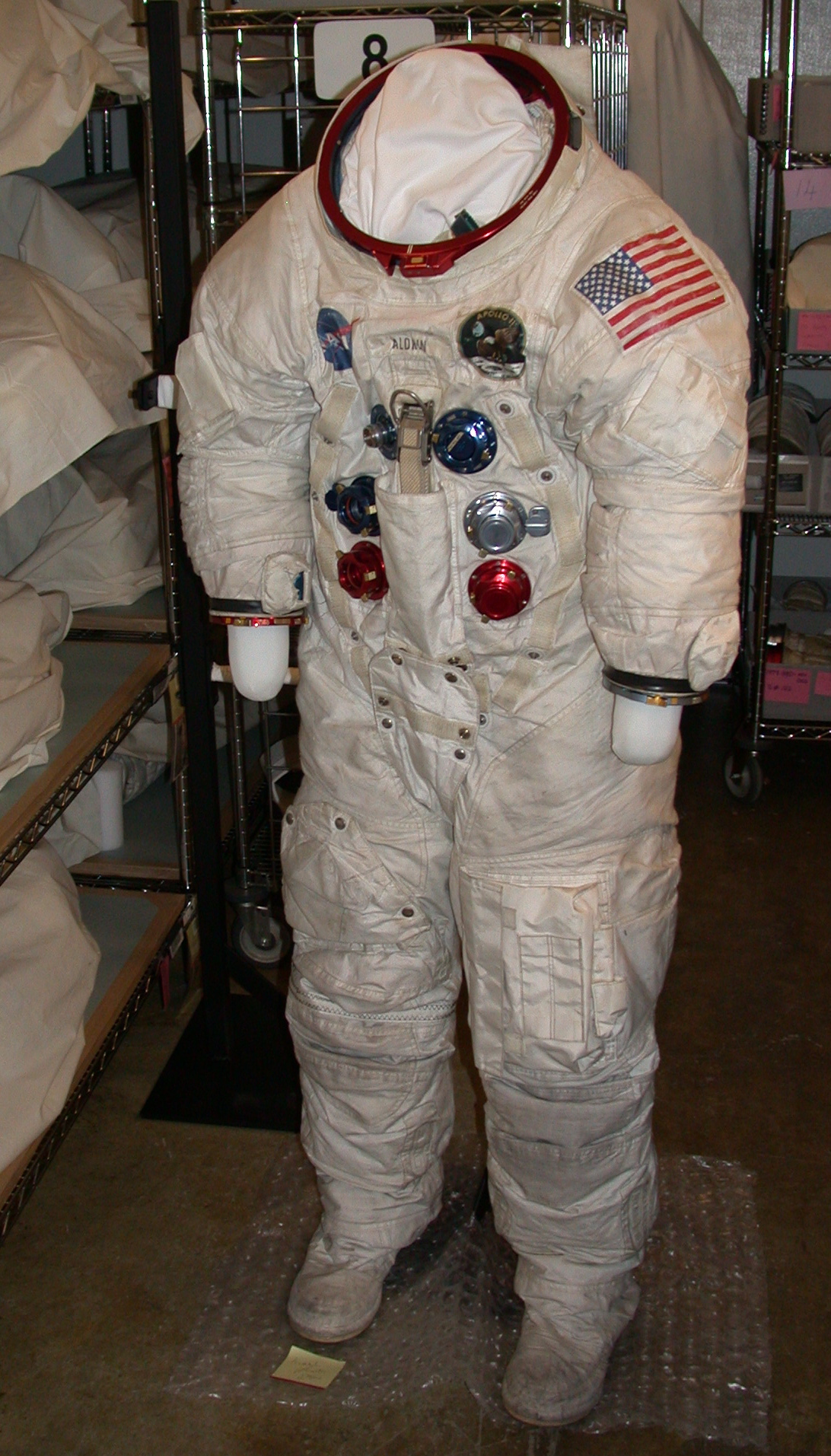The indoor photograph captures a full astronaut's suit displayed on a headless mannequin in what appears to be a storage or warehouse area. The suit is white and puffy but shows signs of heavy use, with brown and gray dirt stains prominently visible. On the left shoulder of the suit, there is a patch of the United States flag, featuring red, white, and blue stripes. The chest of the suit is adorned with several metallic ports and dials of varying colors – two top ones are blue, the middle left is blue, the middle right is silver, and the bottom two are red. A red metal hoop encircles the neck area, which lacks a head, instead covered by a simple white blanket. Between the NASA patch and an Apollo patch on the chest, there seems to be a name, possibly "A-L-O-N-O-N" or "K-O-N".

The suit is situated on a small square of bubble wrap on a solid concrete floor. Surrounding the suit, there are several removable shelves; the ones on the left hold multiple sheets or fabric pieces, possibly covering unseen items, and are fitted with black wheels indicating they are movable. Behind and to the right of the suit, the shelves appear metallic and one bears the label "8" on a white rectangle. A small yellow sticky note is also visible on the floor near the suit.

This detailed composition delineates the environment meticulously, providing insights into the condition and context of the displayed astronaut's suit.